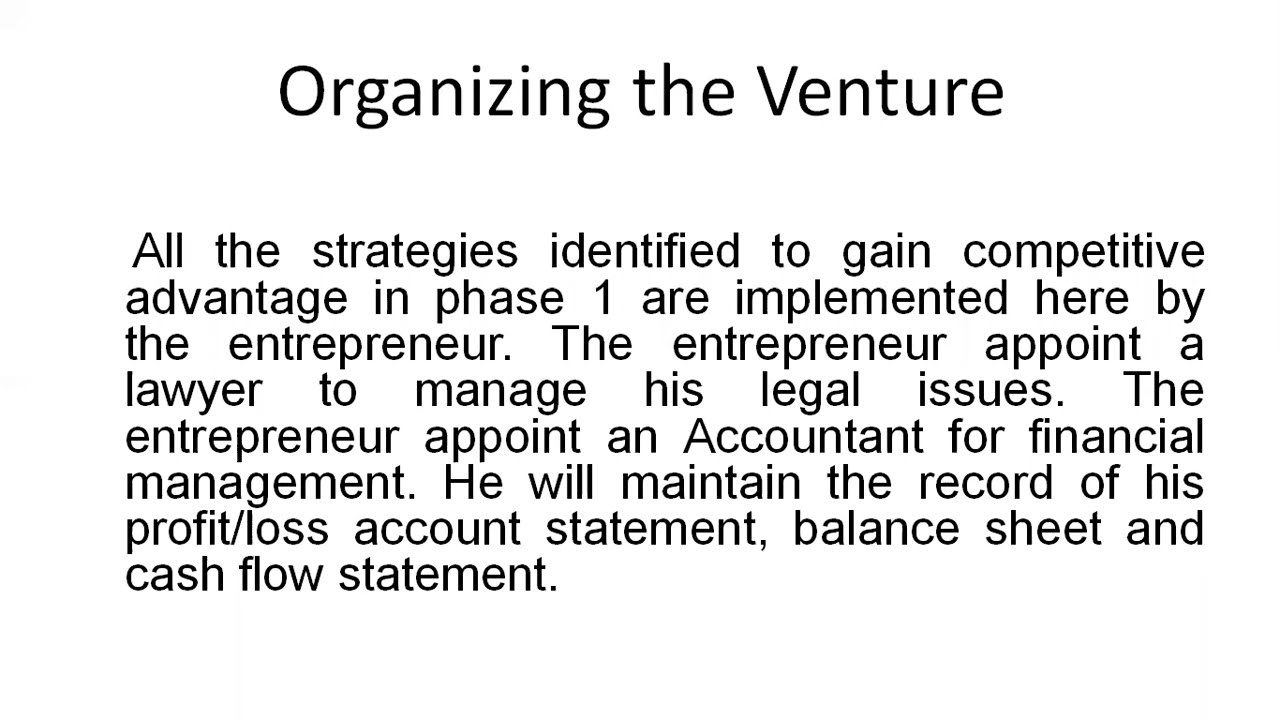The rectangular image features a white background with black sans serif text, resembling a slide from a PowerPoint presentation. Dominating the top in large font is the title, "Organizing the Venture." Below, a detailed paragraph, spanning about seven lines, provides insight into phase one strategies for competitive advantage, which are implemented by the entrepreneur. The text reads: "All the strategies identified to gain competitive advantage in Phase 1 are implemented here by the entrepreneur. The entrepreneur appoints a lawyer to manage his legal issues. The entrepreneur appoints an accountant for financial management. He will maintain the record of his profit/loss account statement, balance sheet, and cash flow statement." Notably, there are several extra spaces between words in the second sentence and a capitalized "Accountant." Although the text is justified, there are some grammatical issues, including missing commas.